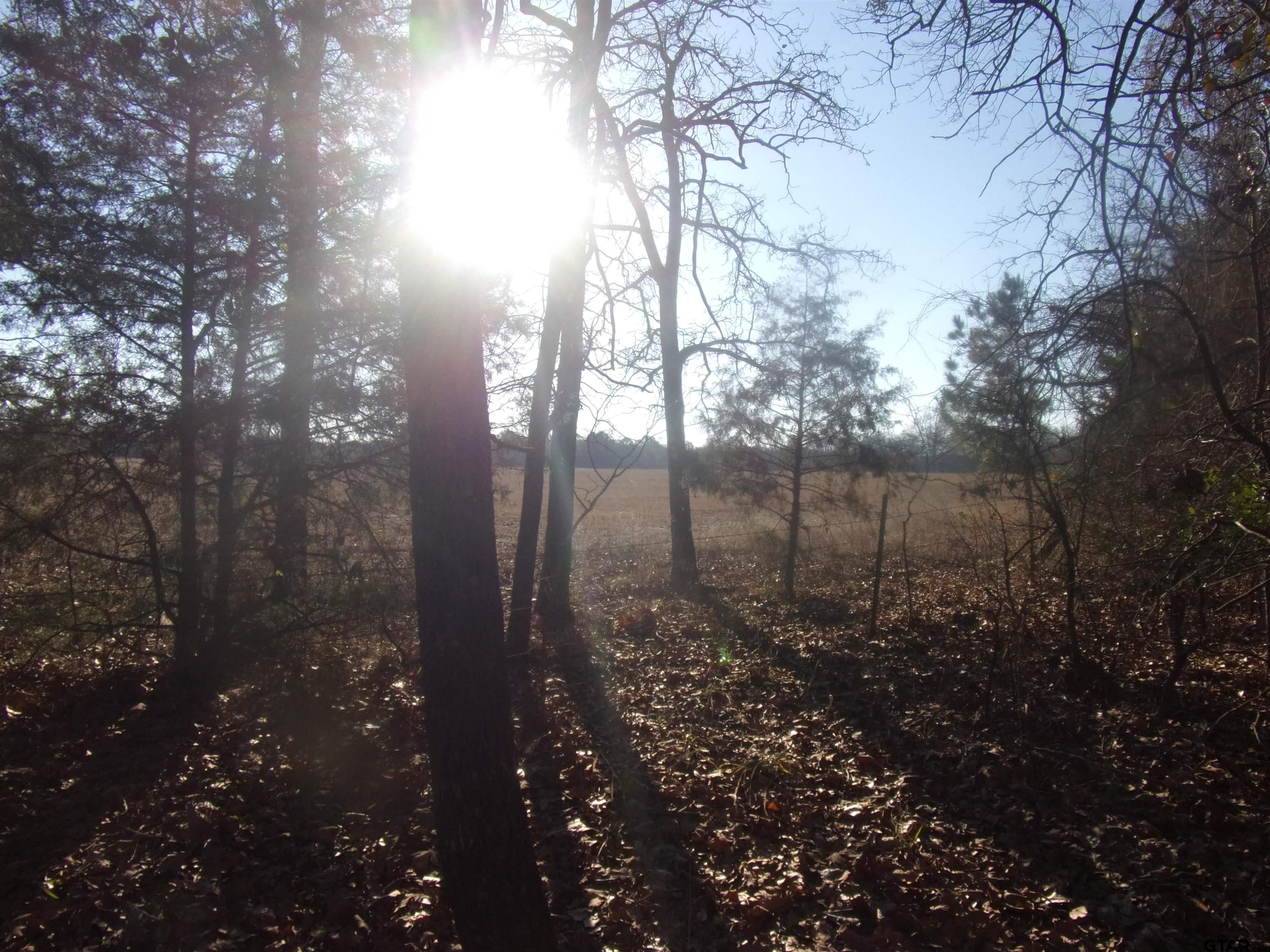As dawn breaks, this captivating early morning photograph captures the serene beauty within a wooded area, looking out onto an open field. The sun's radiant glow filters through the trees, casting a warm, golden light that plays off the leaves, creating long shadows reaching toward the viewer. The sky above is a brilliant, cloudless blue, highlighting the tranquility of the scene. 

The forest floor is a rich carpet of fallen leaves, affirming the season's presence. Near the right edge of the image, young saplings punctuate the space, their small frames contrasting against some evergreen trees, which add vibrant green to the brown and tan palette of the photograph.

Set back about 30 feet into the woods, one can observe a thin wire fence cutting through the middle of the scene, marking the boundary where the dense forest transitions into a vast field of dead, brown grass. This field extends towards the horizon, where another undisturbed patch of forest is visible, and in the far distance, majestic mountains loom under the pristine blue sky.

This harmonious blend of natural elements, with the interplay of light and shadow, the diversity of tree types, and the expansive, untouched landscapes, creates a peaceful and detailed depiction of the woods at daybreak.